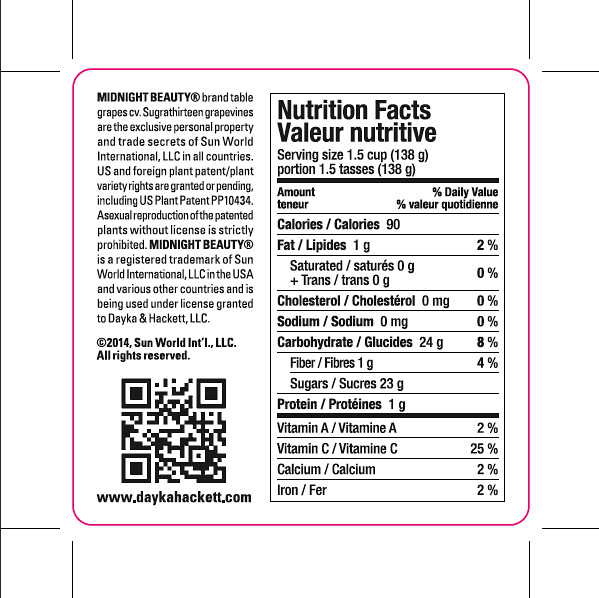The image depicts a detailed nutritional label outlined by a thin pink (or red) line and features possible fold lines marked by short black lines at each corner. The label is for Midnight Beauty Brand Table Grapes, as indicated by the bold text in the upper left, accompanied by a trademark symbol. Below this, a description mentions the exclusivity of the grapes and relevant trade secrets. The right-hand side of the label prominently displays a black-outlined box titled "Nutritional Facts" (or "Valeur Nutritive" in a bilingual format), specifying a serving size of 1.5 cups (138 grams). The nutritional information includes 90 calories, 1 gram of fat, 0 cholesterol, 0 sodium, 24 grams of carbohydrate (8% DV), 4% fiber, 1 gram of protein, 2% vitamin A, 25% vitamin C, 2% calcium, and 2% iron. A QR code is positioned at the bottom left, with the web address www.daykahackett.com underneath.